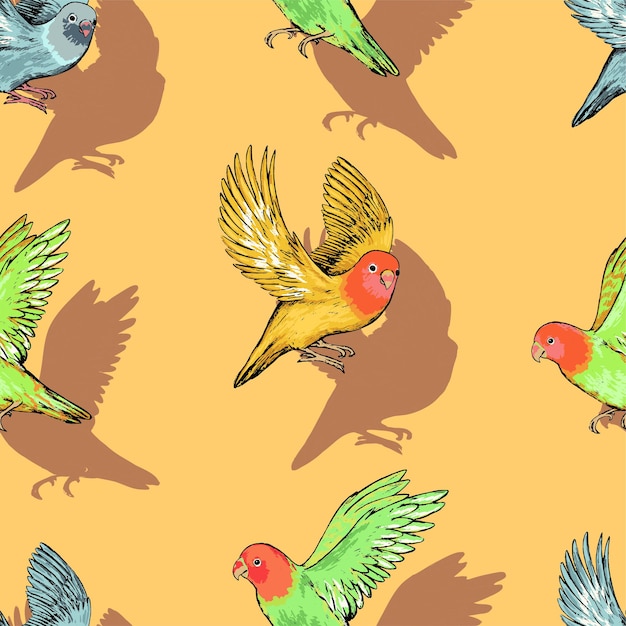This is a detailed digital drawing depicting various types of lovebirds mid-flight, set against a buttercup yellow background. At the center, a yellow and orange lovebird is prominently featured, looking directly at the viewer with its wings outstretched. Surrounding this central bird are several other lovebirds, each partially cropped and casting distinctive black shadows. To the top left, there's a blue lovebird in flight, while in the middle top, only the legs and backside of a green lovebird are visible. To the right, another blue lovebird is seen from the back. Additional lovebirds include a green one with an orange head and a gray-blue lovebird, as well as lovebirds whose blue wings are discernible at the bottom left and right. The birds are evenly spaced, creating a harmonious and colorful composition against the bright yellow palette.